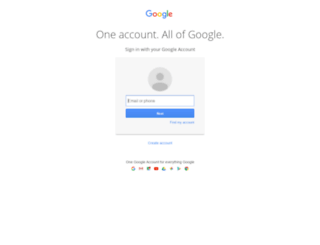This image appears to be a screenshot from a mobile device or a significantly reduced browser window, displaying the Google login page in portrait orientation. At the top of the screenshot, the "Google" logo is prominently featured in its traditional multi-color scheme. Below the logo, in bold black text, the phrase "One account. All of Google" can be seen, followed by "Sign in with your Google Account."

Centered on the page is a light gray square containing a circular icon. Inside this circle is a simplistic gray silhouette of a person, characterized by an oval body and a round head. Directly beneath this icon is a white input field with a blue border, marked with placeholder text that reads "Email or phone."

Below the input field, there is a blue button with white text that says "Next." Further down, there is a faintly visible link, likely reading "Find my account." Outside the gray square, there is a slightly blurry text that seems to say "Create account." Below this, additional text is present but difficult to read, accompanied by various logos representing different Google products. The overall resolution of the screenshot is not very high, making some of the finer details indistinct.